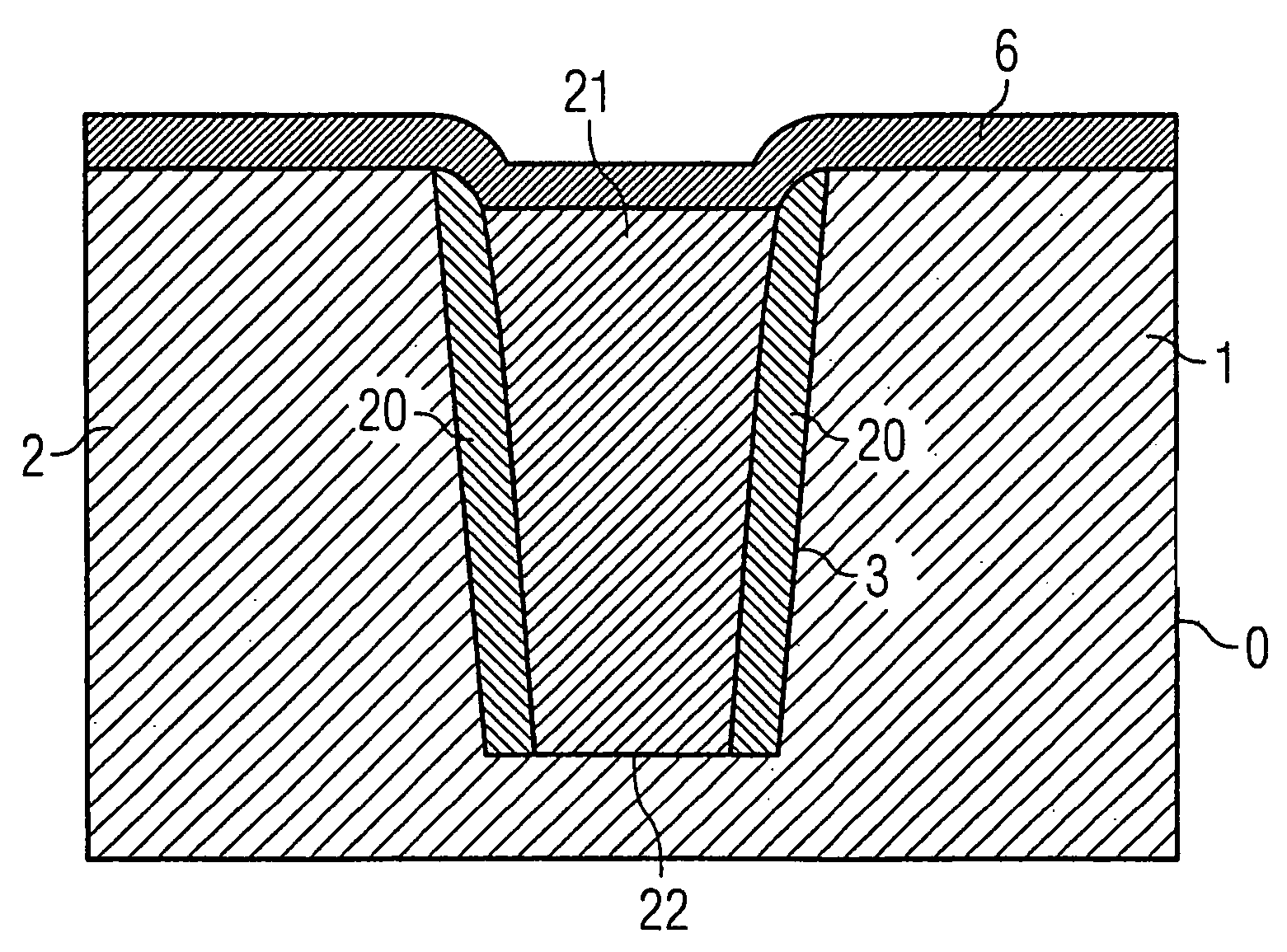This black and white drawing appears to be a technical diagram of a hole or pit set into the ground, possibly designed to hold a pot or other object. The sketch is characterized by a combination of cross-hatched and striped lines, creating varying shades to differentiate parts of the image. At the top of the drawing is a horizontal border marked with closely spaced striped lines indicating a darker, topsoil layer. From this top border, two lines descend, each similarly striped.

The sides of the hole feature wider lines, with the left side having horizontal lines and the right side also marked similarly but annotated with numbers and arrows. The middle of the hole is detailed with closely spaced diagonal lines that run from the top left to the bottom right, while the surrounding ground outside the pit has diagonal lines oriented from the bottom left to the top right. 

The diagram includes several numerical labels: '2' on the left side, '6' at the very top, '21' also at the top, '20' on the left and right sides of the pit, '1' and '0' on the right side, '22' at the bottom, and '23' within the pit. These numbers appear to denote specific points or sections of the diagram, though their exact significance is not immediately clear from the description. The overall effect is a complex, meticulously annotated technical illustration suggesting a specific but unexplained structural design.